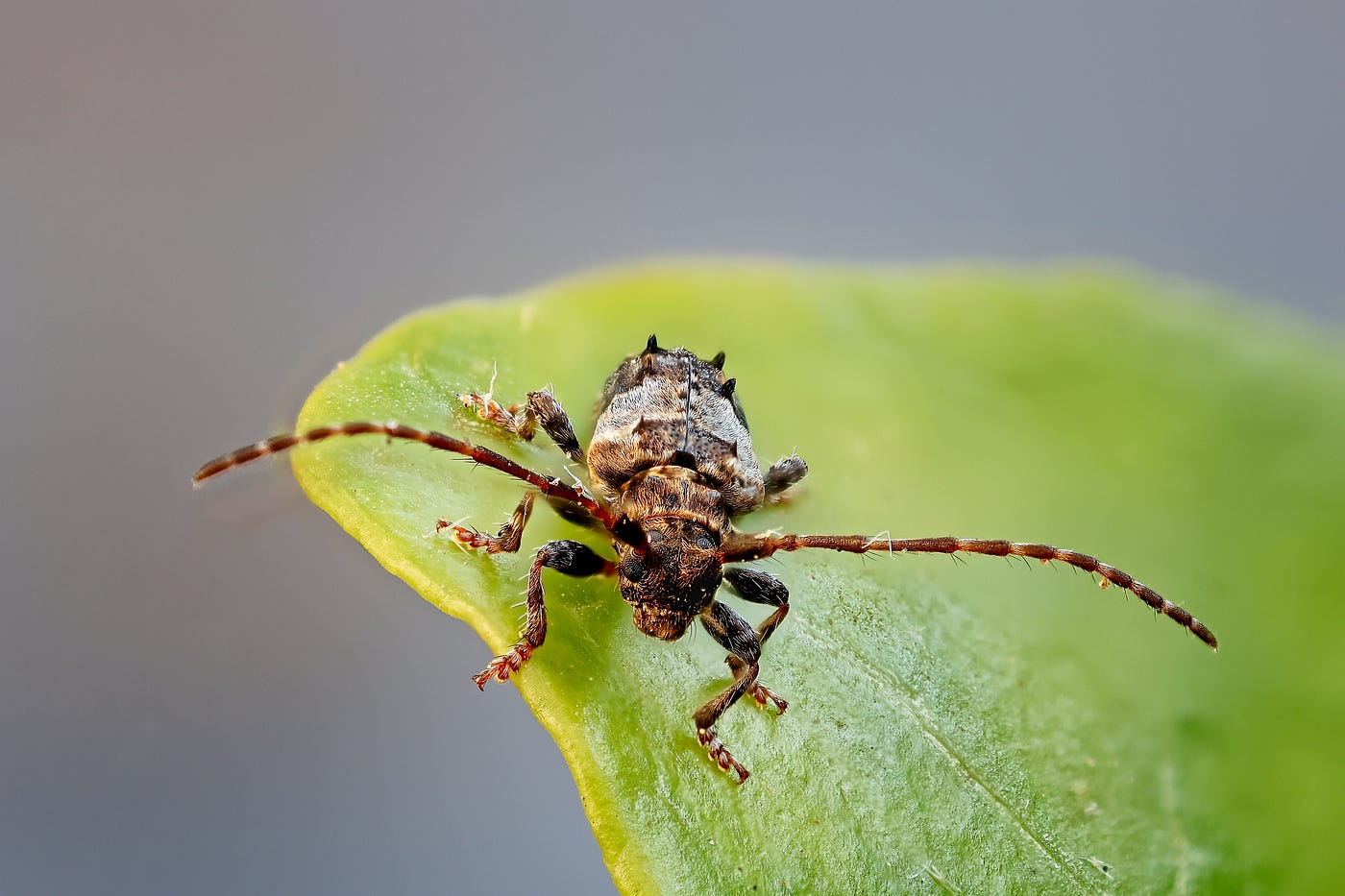The image depicts a close-up view of a beetle perched on a broad, flat green leaf that extends from the right corner, occupying around two-thirds of the horizontal, rectangular frame. The background is a medium gray, providing contrast to the bright green of the leaf. The beetle itself exhibits shades of brown with tan highlights, featuring a strip of tan around its main body. It is adorned with six hairy legs that end in flattened segments, giving the impression of tiny, human-like feet. Two long, hair-covered antennae extend from either side of its head, which appears hard and brown. The beetle's back shows a hard shell with spiny protrusions. One of its feet hangs slightly off the edge of the leaf, while the rest are firmly planted. The beetle appears to be stationary, possibly contemplating its next move under the good lighting that illuminates the scene.